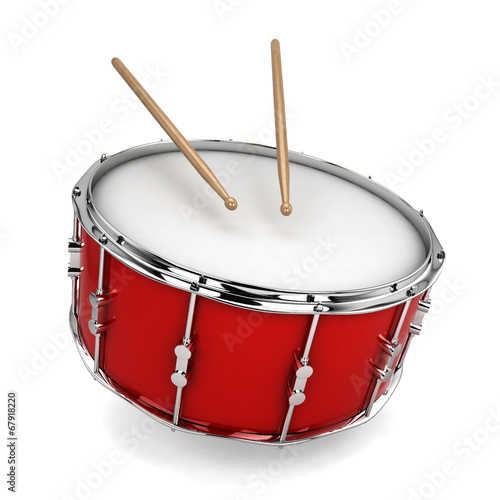The image is a highly detailed 3D rendering of a drum with accompanying drumsticks, set against a clean, solid white background. The red sides of the drum are accentuated by intricate silver vertical metal posts that connect to circular metallic rings encircling both the top and bottom of the drum. The drum's top features a pristine white drumhead, edged with a shiny silver metallic rim. Floating above the drum, there are two light brown wooden drumsticks with rounded, ball-like tips, poised as if ready to strike. The drum, appearing to hover slightly above a flat surface, casts a subtle shadow below, emphasizing its three-dimensional quality. On the bottom left corner, there is black text in a vertical orientation along the side, reading "Adobe Stock number 67918220."